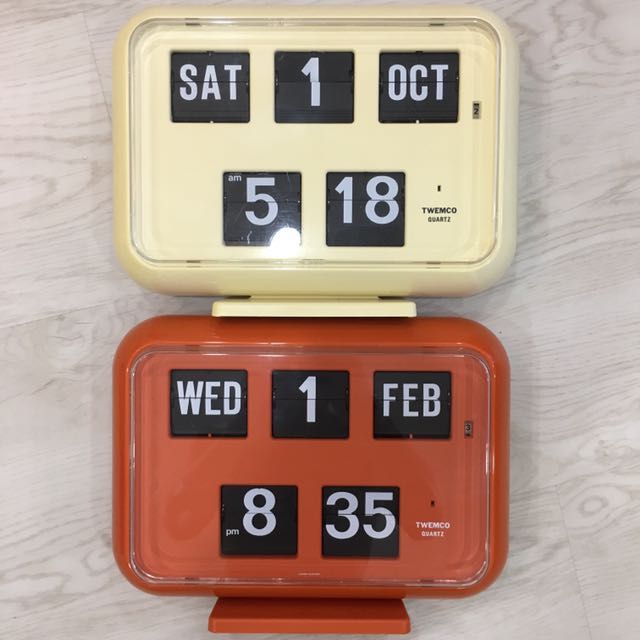The photograph captures two vintage Twemco Quartz digital alarm clocks stacked one on top of the other, set against a light gray, wood-grain background. Both clocks have clear plastic coverings and are identical in design. The top clock is an ivory color and displays the date as Saturday, 1 October, with "SAT," "1," and "OCT" in white over black squares, and the time as 5:18 AM. The bottom clock is orange, showing the date as Wednesday, 1 February, with "WED," "1," and "FEB" in white over black squares, and the time as 8:35 PM.